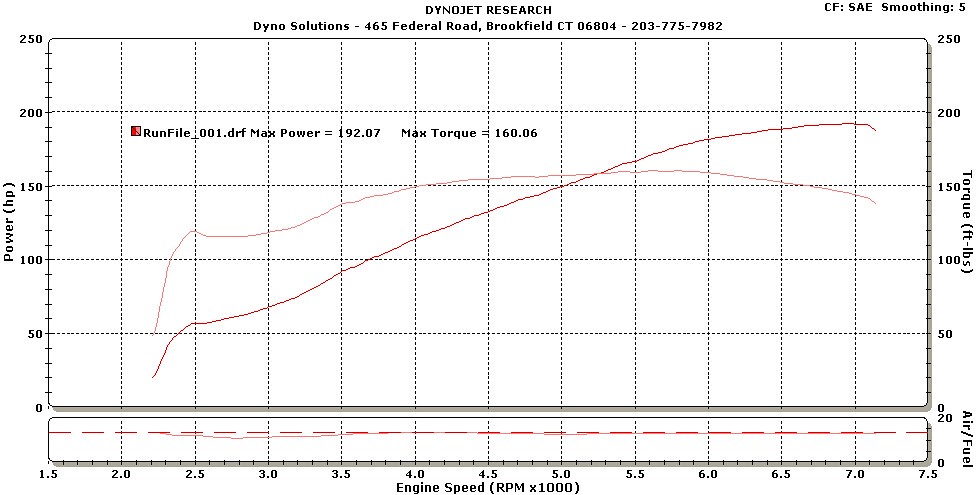This image features a detailed line graph set against a white background with black writing and grid lines creating squares. The graph is titled "Dino Jet Research Dino Solutions" with the address "465 Federal Road, Brookfield, Connecticut 06804" and the phone number "203-775-7982" above it. The y-axis is labeled "Power HP" and displays values ranging from 0 to 250. The x-axis is labeled "Engine Speed rpm x 1000" and ranges from 1.5 to 7.5 in increments of 0.5. The graph includes two distinct lines: a pinkish line ascending diagonally and another line running horizontally. The latter is labeled "run file max torque 160 max power 182."